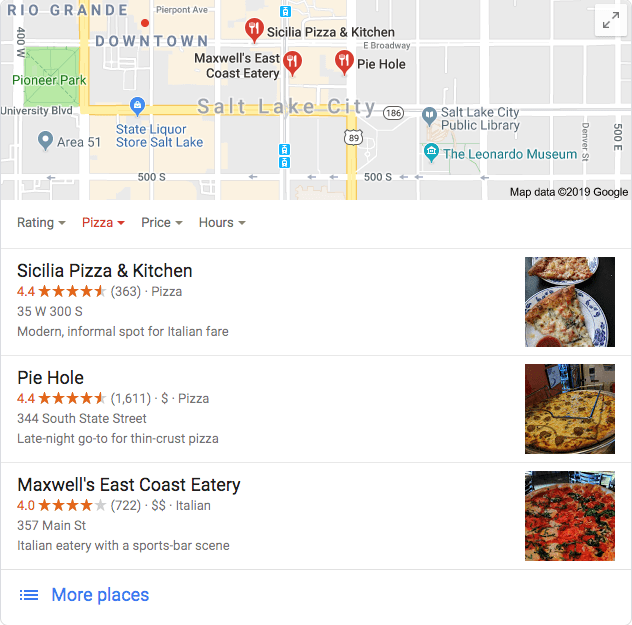The image displays a detailed map highlighting three restaurants in Salt Lake City: Cecilia Pizza and Kitchen, Piehole, and Maxwell East Coast Eatery. The map shows street routes to each restaurant and is marked with key landmarks such as Pioneer Park, the downtown area, Salt Lake City Public Library, and the Leonardo Museum. The top part of the image features the map with these highlighted locations, providing a comprehensive view of the area.

Each restaurant is detailed with specific ratings, categories, price ranges, and hours of operation. Cecilia Pizza and Kitchen, located at 35 West 300 S, has a rating of 4.4 stars. Piehole, situated at 344 South State Street, also boasts a 4.4-star rating. Maxwell East Coast Eatery, found at 357 Main Street, carries a 4.0-star rating. The image serves both as a geographical guide and a review summary for potential diners looking to explore the pizza options in Salt Lake City.